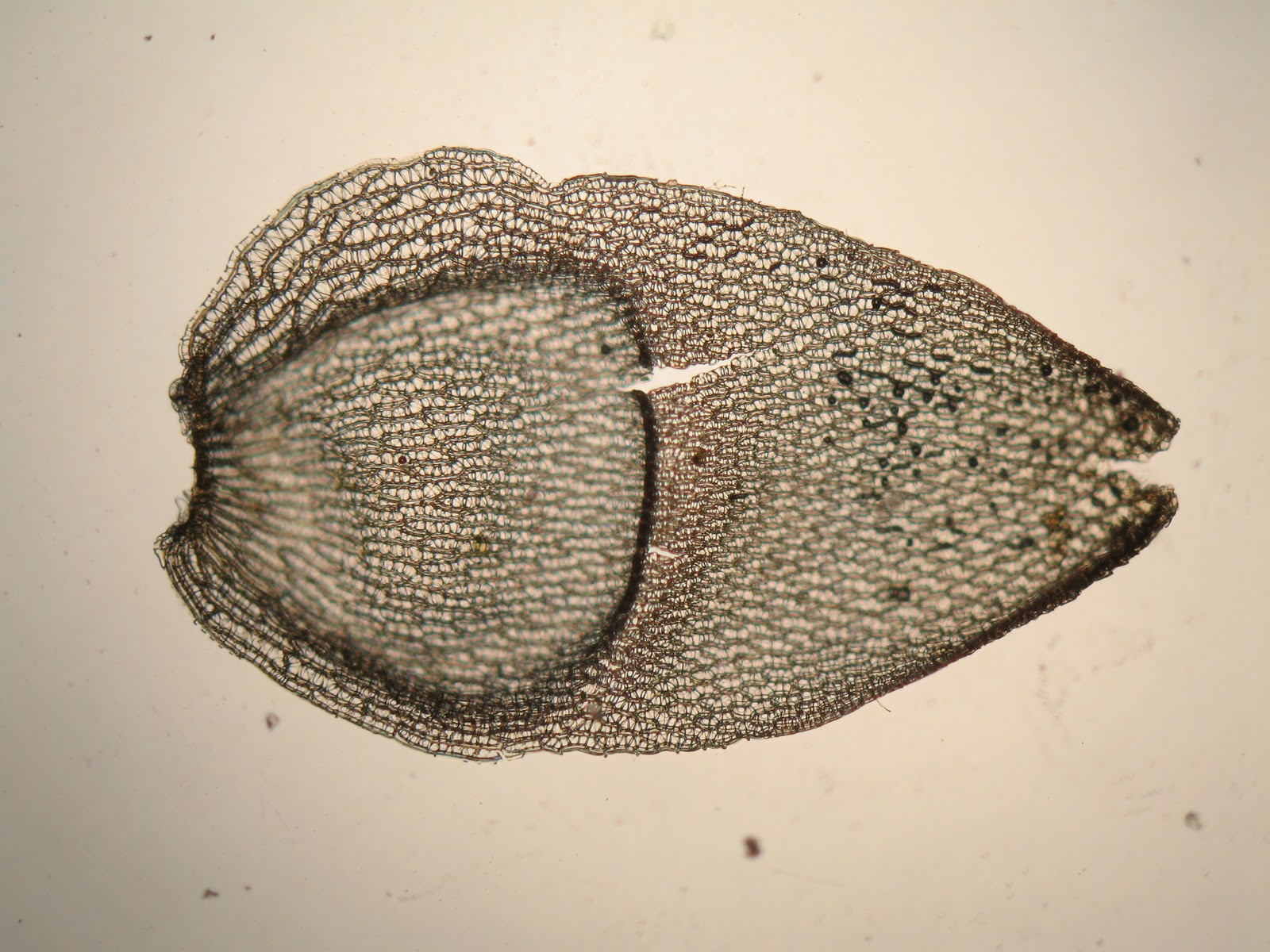This detailed image captures a microscopic view of a single-celled organism with an egg-shaped, brown-colored body. The organism appears to be oriented sideways; at its front side, a large vacuole is clearly visible. The darker brown color highlights both its mouth and tail areas, contrasting with the rest of the body. The background of the image features a light gray and light lavender hue, decorated with scattered black and brown spots. The image composition is framed within a square, and the overall aesthetic suggests intricate details akin to woven patterns, indicating finely indented lines and white spots.